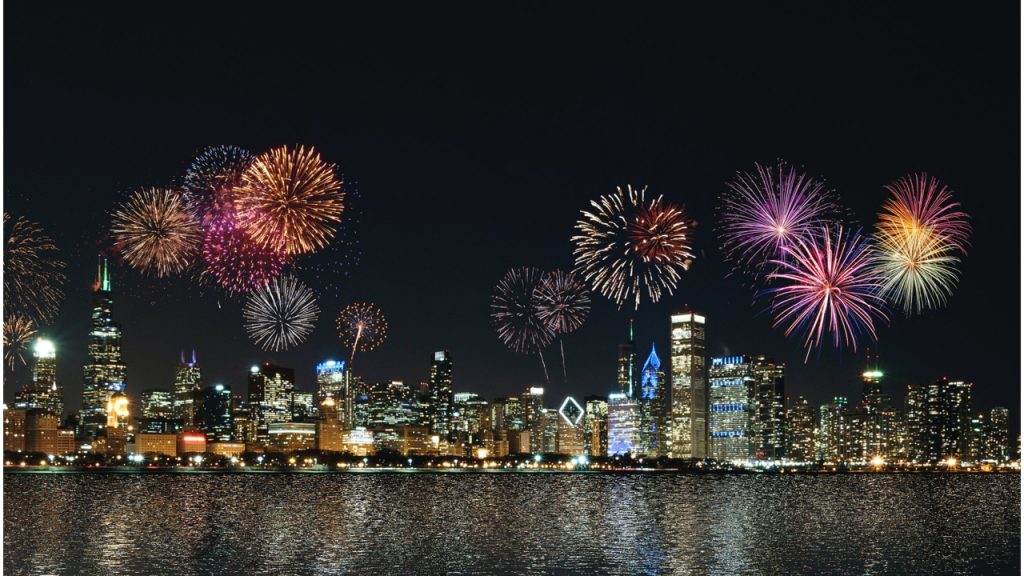The image captures a vibrant nighttime firework display over a bustling city skyline, possibly New York or Hong Kong, viewed from across a river or harbor. In the foreground, the dark water reflects the colorful bursts, creating a shimmering, blurred array of hues. The background features a dense cityscape with a range of skyscrapers—some towering, others short, illuminated with an assortment of blue, yellow, and white lights. Notable is a distinctly triangular building on the left side among the standard rectangular structures. The fireworks explode in a glorious array of colors including yellow, purple, pink, white, and orange, their patterns resembling sunflowers as they burst and scatter skyward, adding a festive, dynamic element to the serene, dark sky.